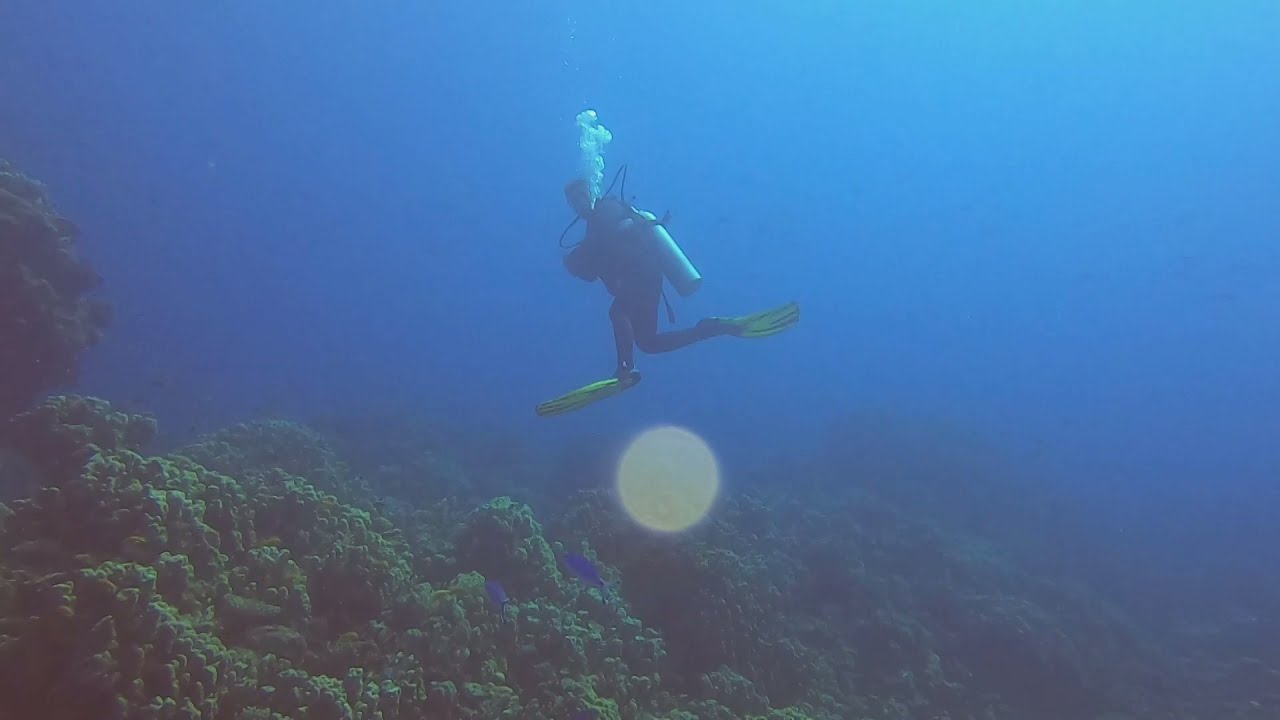A color photograph in landscape orientation captures a lone scuba diver approximately 30 yards from the viewer, centered in the deep blue gradient of the ocean. The diver, adorned in a black wetsuit and yellow flippers, carries a silver oxygen tank on their back. A stream of bubbles trails from their breathing apparatus into the surrounding murky, yet clean waters. The ocean floor, primarily visible in the bottom left foreground, is covered in a moss-like coral with varying shades of green, including dull yellowish-green patches. The vibrant blue of the ocean deepens to a darker hue as it extends into the background, devoid of fish, except for a few smaller ones subtly noticeable near the coral. A possible lens glare effect, resembling a circle, is seen beneath the diver, adding an additional point of interest to the underwater realism of the scene.